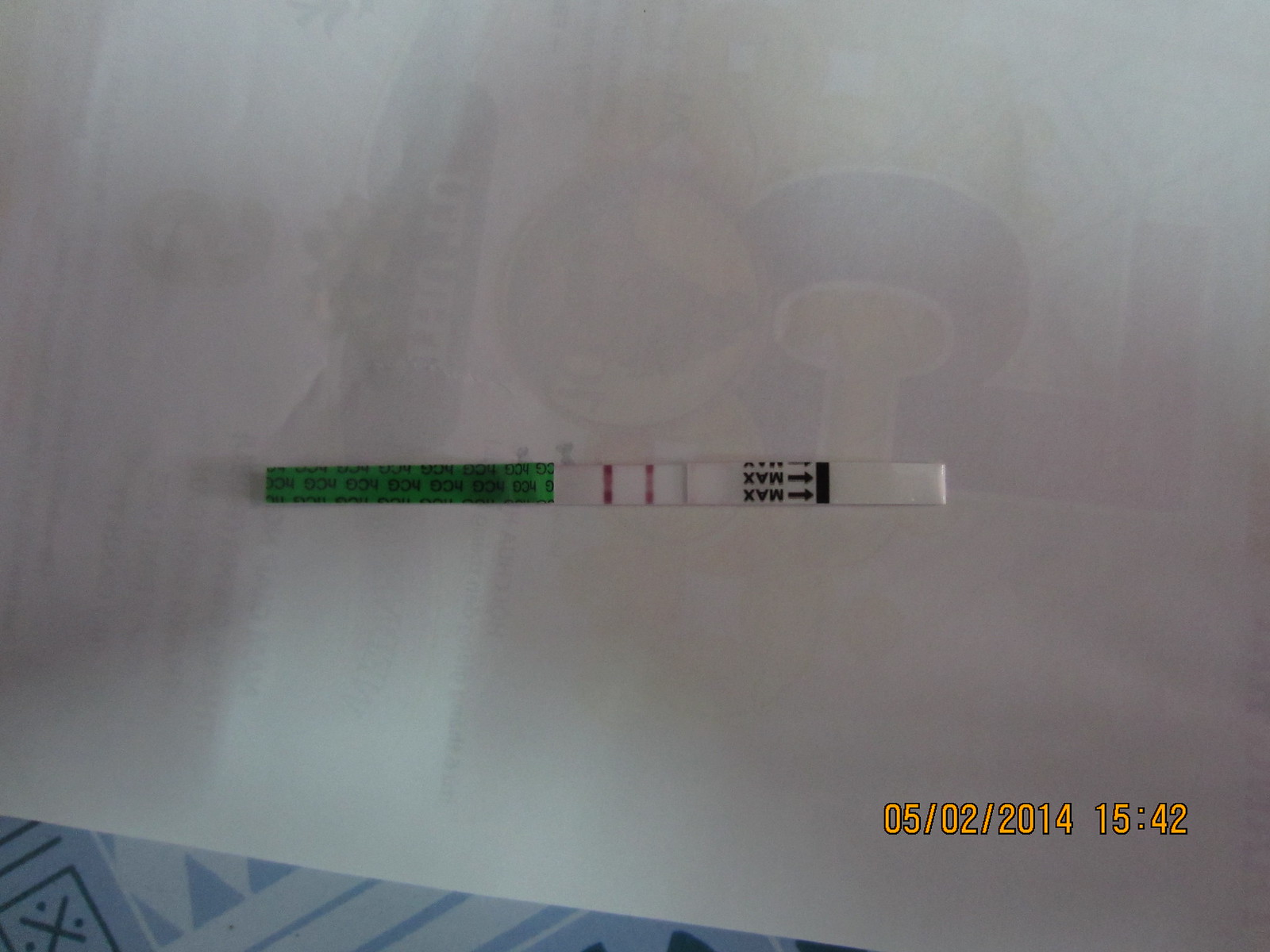In the bottom right corner of the image, displayed in yellow text, is the date "05/02/2014" followed by the time "15:42". The image prominently features a white piece of paper, the details of which are not entirely discernible, but it appears to be the back of a printed sheet. Although the text on the paper is partially visible and indecipherable, one can vaguely make out the letters "UTUHT" and perhaps a backwards "C" above an "L", accompanied by an illustration that resembles a globe.

The primary focus of the image is a thin, white test strip placed on top of the paper. The test strip itself is predominantly white with a green section on the far left side, which displays indistinct letters that seem to spell "NCG." Along the length of the strip, two red lines are visible, and the word "MAX" is printed twice in black, albeit upside down. Additionally, there are two black arrows pointing at a black line on the strip.